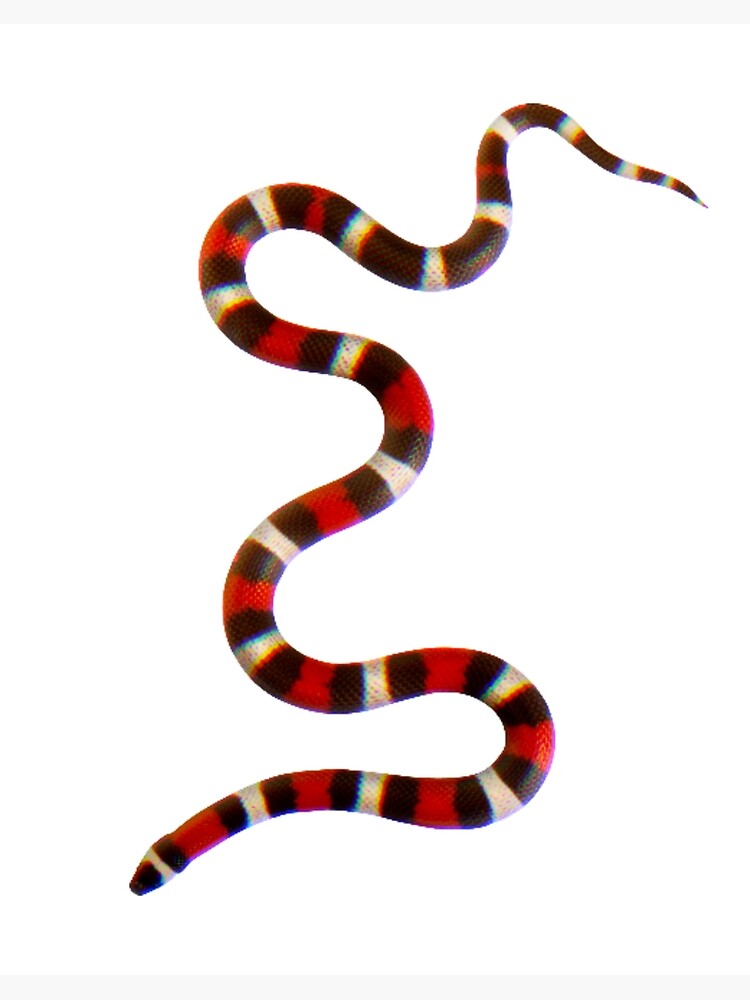This is a highly detailed, computer-generated color image featuring a single snake. The serpentine creature is depicted in a graceful, sinuous curve that spans the entire image, with its head positioned at the bottom left corner and its tail extending to the top right corner. The snake's body is adorned with striking stripes that follow a pattern of alternating colors: red, black, white, black, red, and so on, continuing to the very tip of its tail. Set against a pristine, solid white background, this vividly colored snake is the sole focus of the image. The composition is minimalistic, with no additional elements such as text, other animals, people, plants, or buildings, allowing the viewer to fully appreciate the intricate design and vibrant coloration of the snake.